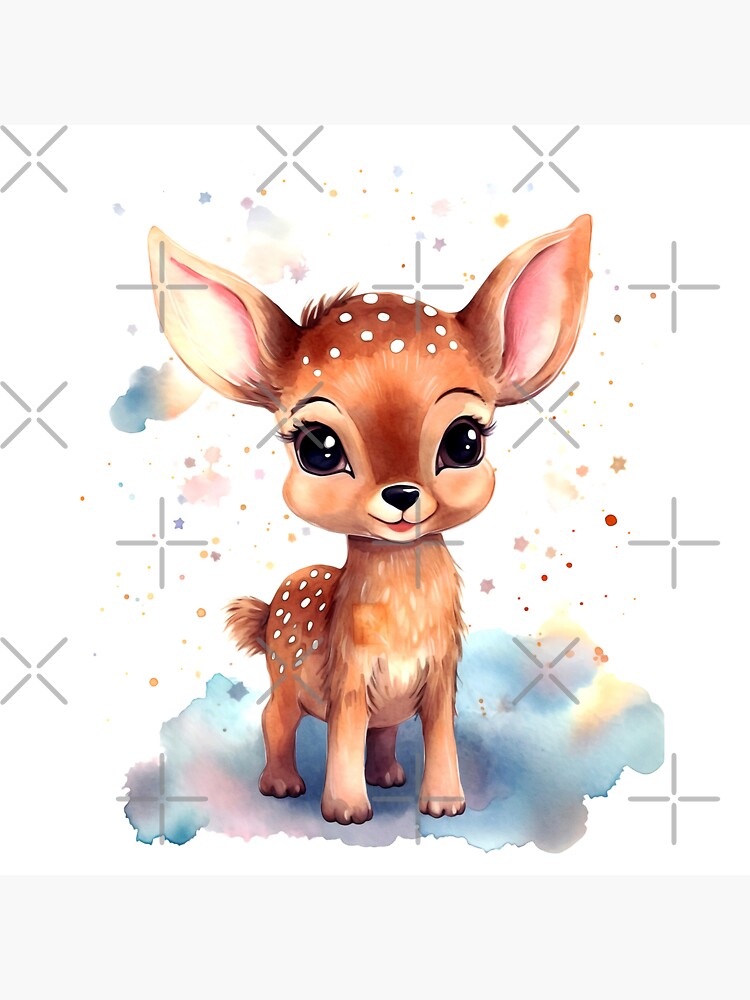The image is a watercolor painting of an adorable baby fawn deer, depicted in a whimsical and vibrant style. The deer, with its wide, expressive doe eyes, looks happily towards the viewer. Its large head is adorned with delicate white spots, which are also scattered along its back. The fawn's soft brown fur contrasts with the pinkish interior of its large ears, and it has long black lashes and a little black nose. Its tiny bushy tail complements its overall cute appearance. The deer stands atop a colorful, dreamy cloud predominantly in shades of blue, with hints of purple, white, yellow, and a subtle black-purple. The background features additional watercolor splashes and marks, interspersed with playful X's and plus signs, and sprinkled with dots in pinks, blues, and yellows. The overall composition gives a dreamy, fairy-tale quality to the painting, enhancing the charm of the wide-eyed, serene fawn.